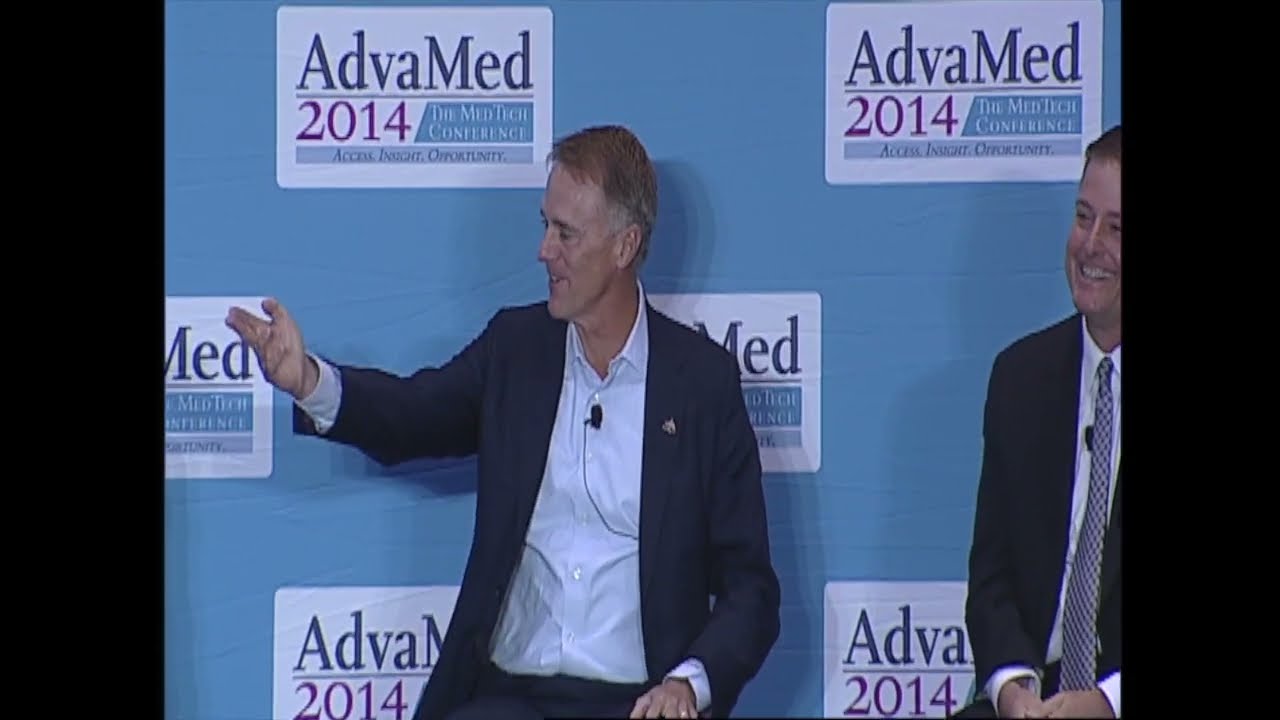The image features a man at a press conference, implied by the blue brick wall backdrop adorned with repeated white signs that read "2014 The MedTech Conference: Access Insight Opportunity." He is dressed formally in a black suit jacket, paired with a white collared shirt and a dark checkered tie. A small microphone is clipped to his tie or shirt. His hands are outstretched in front of him with palms facing inward, and his eyes are half-closed. The man has short hair, fair skin, and a gold wedding band on his fourth finger. The setting suggests he is possibly speaking on a panel, as light in front of him casts shadows on the stage, and a partial view of another individual is visible to his left.